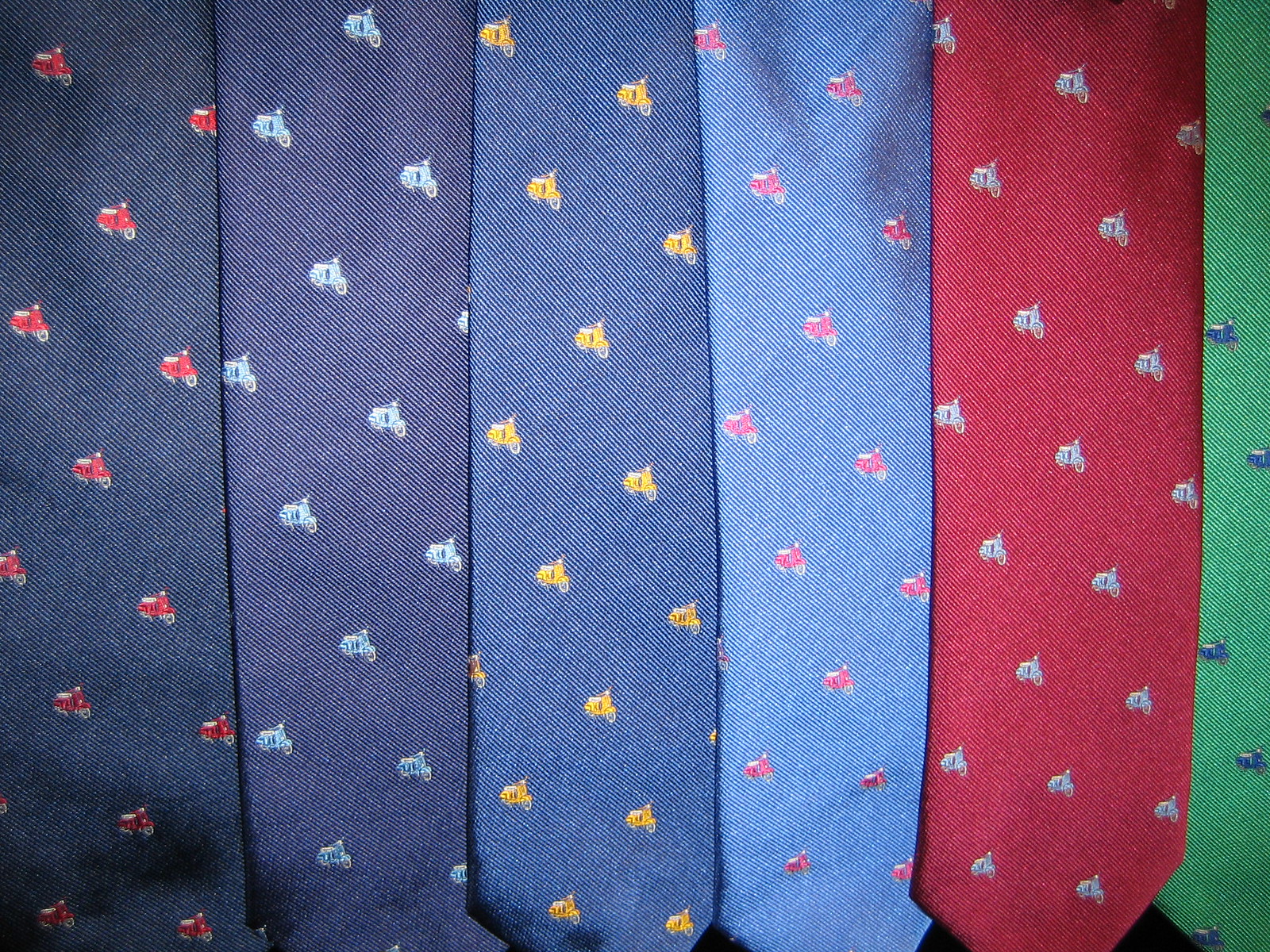This detailed image features an extreme close-up of six different neckties arrayed side by side against a black background that peeks through the gaps. Each tie is distinct in color and pattern but shares a common motif resembling small wagon-like or train head designs. From left to right, the ties are as follows: 

1. A dark blue tie adorned with small red wagon-like patterns. 
2. A purplish tie with light blue wagon-like patterns. 
3. A navy blue tie featuring yellow wagon-like designs. 
4. A lighter blue tie with pink wagon-like patterns.
5. A red tie decorated with gray wagon-like patterns.
6. A green tie with dark blue wagon-like patterns.

The ties appear to be hanged and the image captures only their lower portions, emphasizing the intricate patterns and color variations.